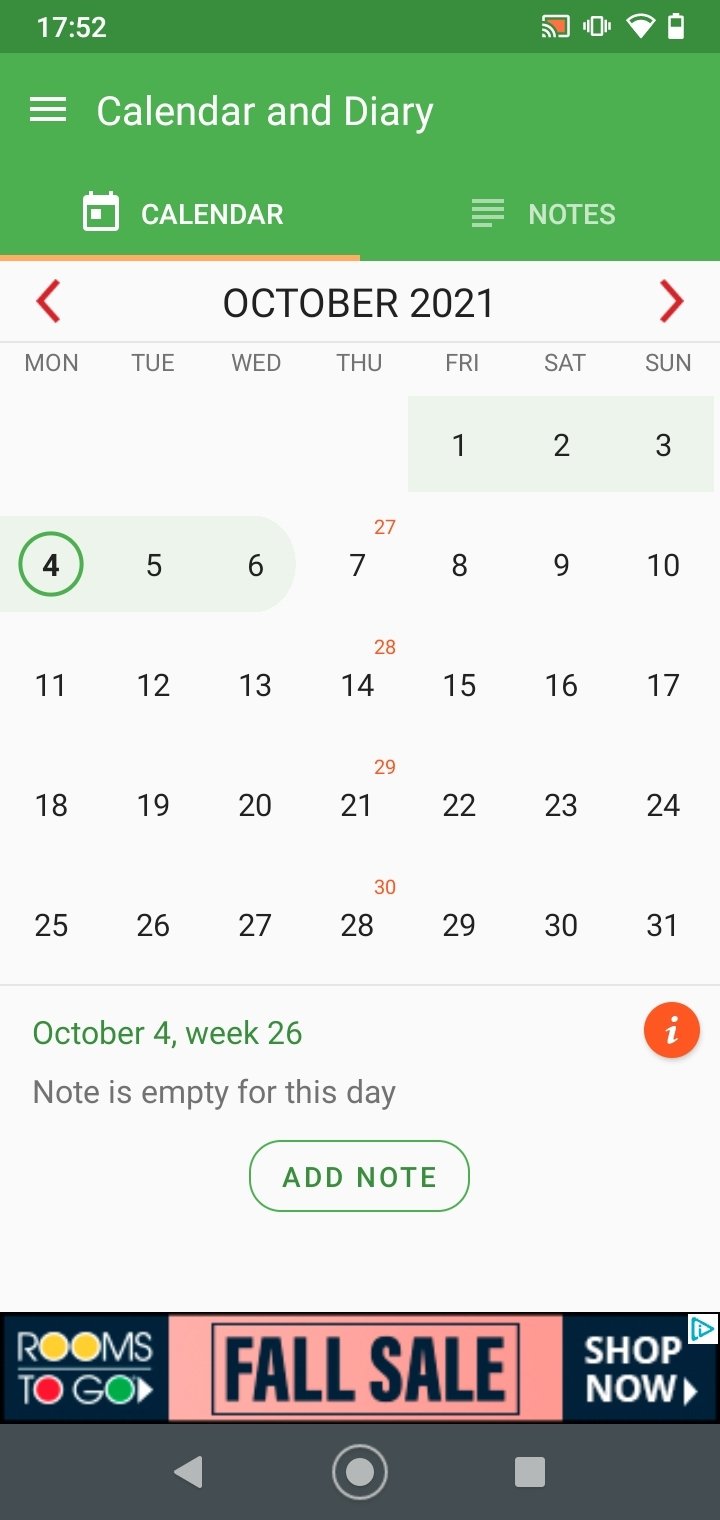**Detailed Caption:**

The image is a screenshot of a mobile phone displaying a calendar application in portrait mode, specifically showing the month of October 2021. The top portion of the screen features a green background title reading "Calendar and Diary," with two tabs below labeled "Calendar" and "Notes." 

In the calendar view for October 2021, the month begins on a Friday (October 1st) and ends on a Sunday (October 31st). The dates from October 1st to October 6th are highlighted in gray, with Monday, October 4th distinctly circled in green. Below the calendar grid, it is noted as "October 4th, Week 26," indicating that no note has been added for this day, although there is an option available to add one.

Among the days listed, the Thursdays stand out as each has a red number in the upper-right corner of the date box. Specifically, Thursday the 7th has the number 27, Thursday the 14th has the number 28, Thursday the 21st has the number 29, and Thursday the 28th has the number 30.

At the bottom of the screen, an overlay ad for "Rooms To Go" is visible, promoting a fall sale, which is typical for the application.